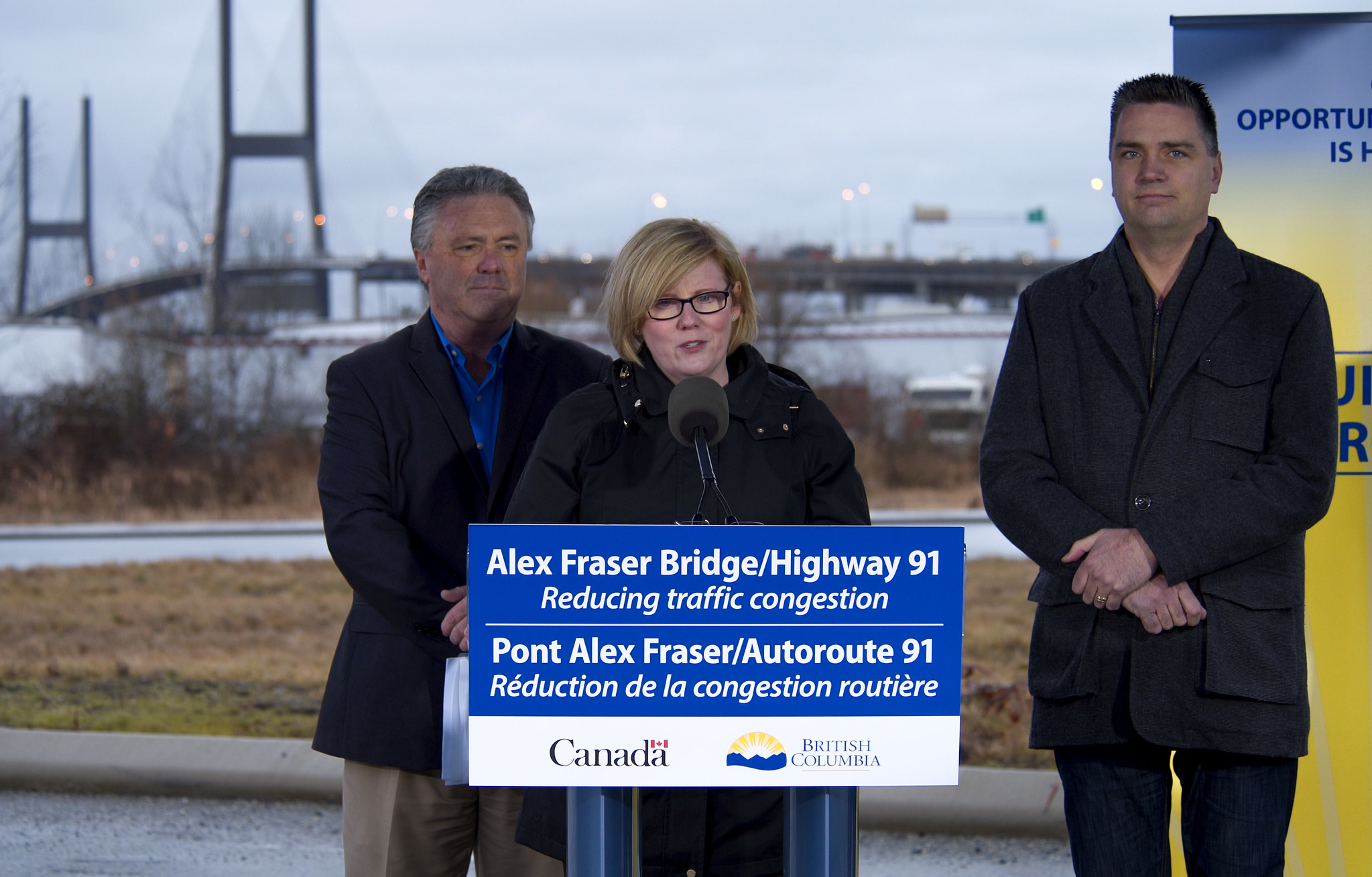In this outdoor scene, a woman with short blonde hair and glasses stands behind a podium, delivering a speech into a large black microphone. She is dressed in a black jacket and positioned in front of her is a large rectangular poster that reads "Alex Fraser Bridge, Highway 91, Reducing Traffic Congestion," also translated into French, indicating that this is in British Columbia, Canada. Flanking her are two men: to her left, a man with short black hair wearing a black sports jacket and tan pants, and to her right, a taller man with short black hair dressed in a black jacket and pants. Both men stand with their hands folded in front of them, observing the proceedings. The background reveals an outdoor setting with an expansive bridge, a beige landscape, patches of grass, trees, and a gray sky, suggesting a formal announcement related to the highway's efforts to alleviate traffic congestion.